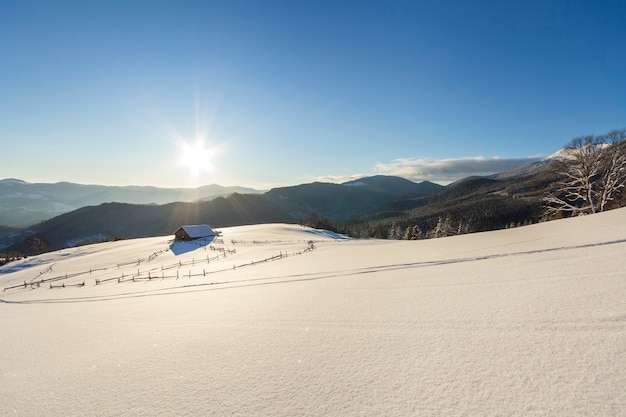A picturesque scene depicts a solitary wooden cabin nestled in a snow-covered field, surrounded by a short wooden fence. The cabin, longer than it is wide, rests on a gentle incline with snow reaching up to its roof in the back. The landscape is set in a mountainous forest area during winter, with the snow blanketing the ground and the cabin’s roof. In the middle ground to the left of the image, the cabin stands out prominently, while a few barren trees with snow-dusted branches surround it. The sky above is a nearly clear blue, except for a small patch of clouds over the snow-clear mountains on the right side. The rising sun shines brightly, casting gleaming rays over the scene, creating a serene and luminous atmosphere. Far-off on both sides, mountain ranges stretch into the distance, with thick forests covering their slopes, contributing to the secluded and tranquil setting of this alpine haven.